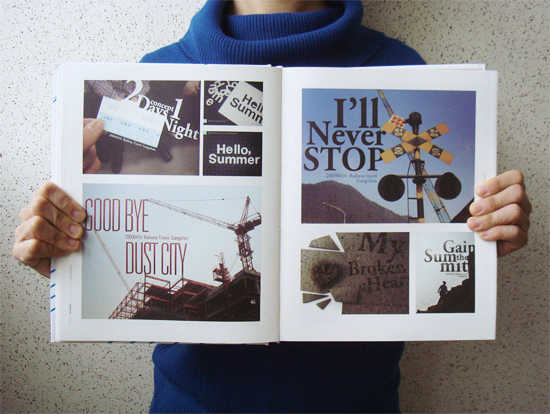The image showcases a person wearing a blue turtleneck, partially obscured by an open book they are holding. Only their hands and the upper part of their neck are visible, making it difficult to ascertain their gender. The background features a white or off-white wall with specks that are part of the design. The book appears to be a scrapbook or photo album, filled with various photographs and captions. 

On the left page, the captions read "Hello Summer" at the top, followed by "Two Days, One Night." Below this is a picture of a construction site with a crane, labeled "Goodbye Dust City" in red. The right page features a sky-blue background with a train stop and the caption "I'll Never Stop" in black. Additional images include a person climbing a mountain with the phrase "Gain the Summit" at the bottom. The photographs are mostly subdued in color, except for the bright blue sky and yellow railroad crossing, which stand out. This scrapbook likely documents a summer celebration or vacation, capturing various memorable experiences.